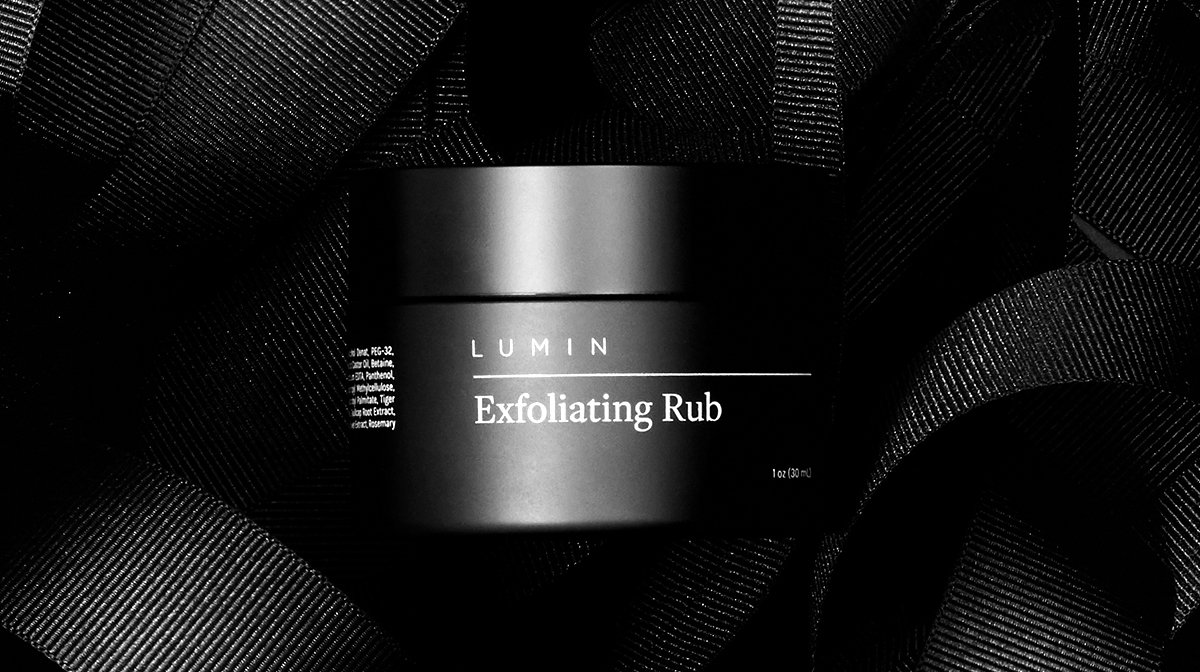The image is a horizontal rectangle with a primarily black background, featuring shades of gray and textured elements that resemble black straps, akin to those found on backpacks or suitcases. These straps are arranged in various positions; some are tightly close together while others are curved or hanging loosely, adding a graphic design effect. Central to the image is a black, cylindrical jar typically used for cosmetics. The jar displays a label with the brand name "LUMIN" in white text at the top, followed by a thin horizontal line. Beneath the line, in larger, bolder white text, the label reads "Exfoliating Rub." To the left, there is small, fine print which might list ingredients, although this part is partially cropped. Additionally, at the bottom right of the jar, very small white text indicates the product's volume: one ounce or 30 milliliters.